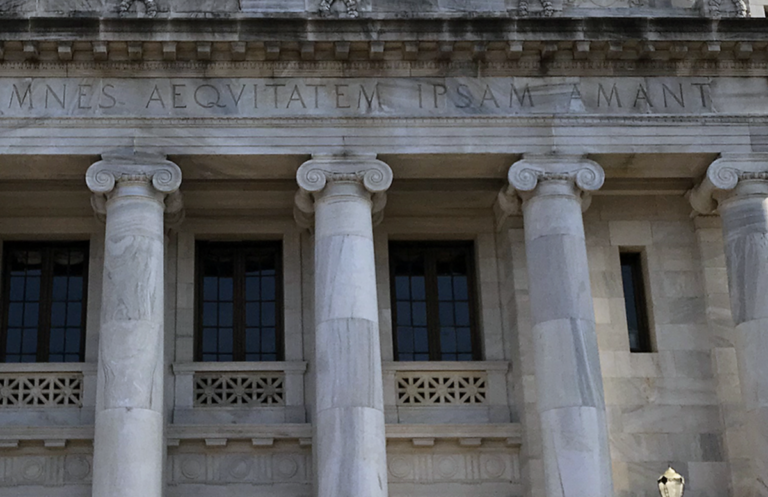This image captures the front of a dignified, old-fashioned building reminiscent of the architectural style seen in the United States Capitol or the White House in Washington, D.C. The structure, constructed from large white marble or granite bricks, features four imposing round pillars at its façade, complete with ornate curls at their capitals. The top of the building boasts an inscription in Latin, "AEQUITATEM IPSAM AMANT," which translates to "they love equality itself." Below the inscription are three Juliet balconies, lending an artistic touch rather than serving as functional spaces. These mock balconies are positioned in front of tall, double-paned windows that tilt slightly to the left in the image. An additional long, narrow window can be seen to the far right. The building exudes a somber elegance, characterized by its ornate designs and dark, muted gray tones.